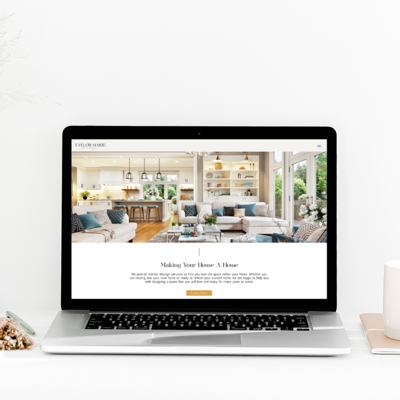This image depicts a modern living room seamlessly integrating with an open kitchen area in the background. Dominating the foreground is a screenshot of a sleek notebook or laptop, featuring a silver body and black keys, with a webpage displayed on the screen. The living room furniture includes pristine white couches adorned with vibrant, multi-colored pillows in shades of white, blue, and black. Overhead lamps illuminate the kitchen’s bar area, which is equipped with contemporary bar stools.

To the right, a door leads out to an outdoor area or deck, inviting natural light into the room. Close examination reveals a decorative element with the slogan "Making Your House a Home" accompanied by a yellow button, though its details are partially obscured. On the bottom left of the screenshot, there appears to be an array of walnuts or similar items. Additionally, a notepad and either a coffee cup or an Alexa device are visible, adding to the cozy ambiance of the scene.

The webpage displayed on the laptop is largely indiscernible, contributing to the casual yet sophisticated atmosphere captured in this home setting.